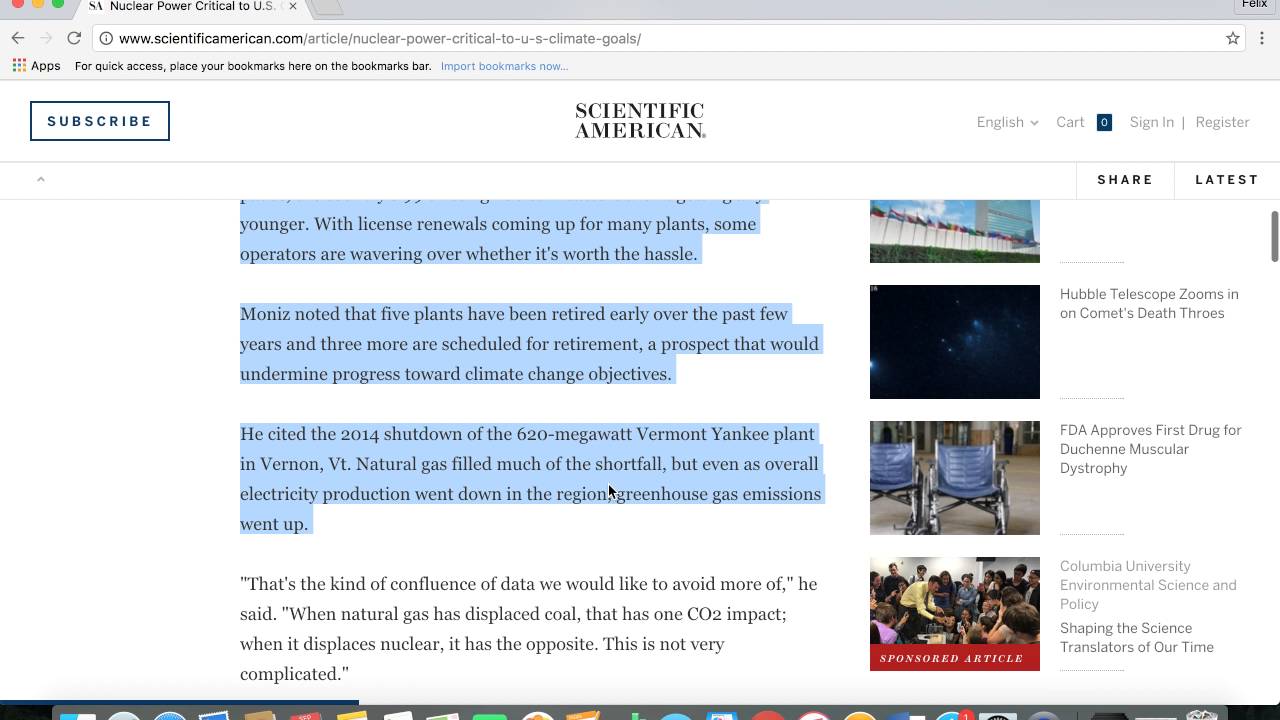The screenshot from Scientific American depicts an article highlighting the importance of nuclear power for the U.S. climate goals. The URL at the top ends with "article/nuclear-power-critical-to-U.S.-climate-goals." On the left side of the page, there is a prominent "Subscribe" button, while on the right, options for "English," "Cart (0)," "Sign In," and "Register" can be seen. The article text, set within a blue-highlighted background, discusses the debate over nuclear plant license renewals. It mentions that several operators are reconsidering the worth of renewing licenses due to the hassle involved. The text specifically states that five plants were retired early in recent years, with three more scheduled for shutdown, a move that could hinder climate change mitigation efforts. It references the 2014 shutdown of the 620-megawatt Vermont Yankee plant in Vernon, Vermont, noting that while natural gas compensated for some of the lost electricity, overall greenhouse gas emissions increased even as electricity production in the region decreased.